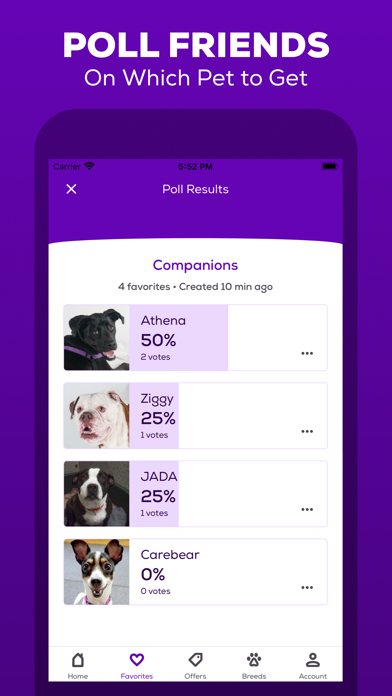This image displays a screenshot of an app called "Poll Friends." At the top, the app's title is clearly visible, followed by the poll question, "On which pet to get?" The poll results are shown beneath, presented in a structured format. The poll, which was created 10 minutes ago, has the following results:

- Athena: 50% with 2 votes
- Ziggy: 25% with 1 vote
- Jada: 25% with 1 vote
- Care Bear: 0% with 0 votes

At the bottom of the screen, there is a navigation bar with tabs labeled "Favorites," "Offers," "Account," "Breeds," and "Home," allowing users to easily explore different sections of the app.